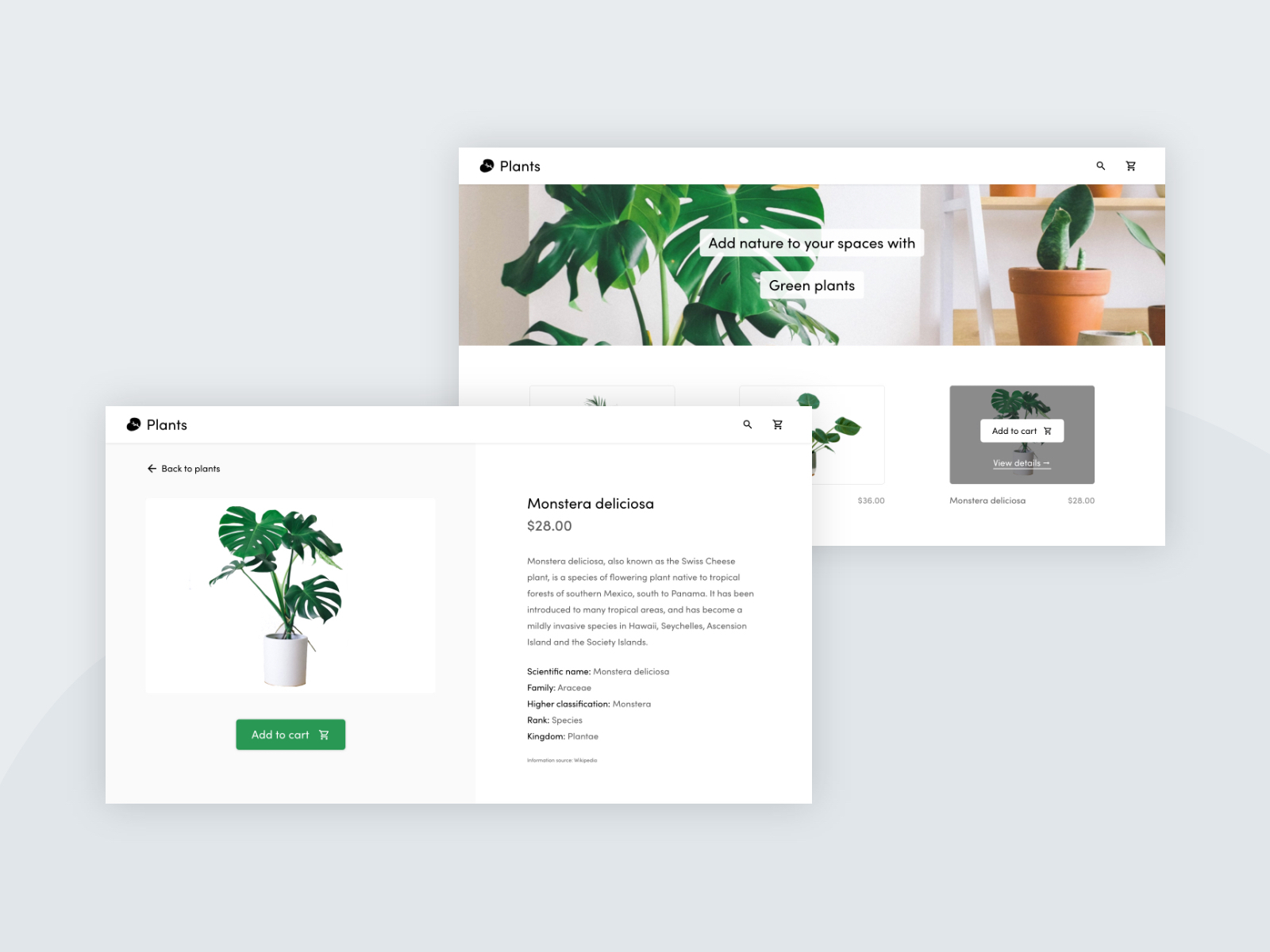In this visually appealing image set against a light gray background, two white rectangular boxes overlay each other, showcasing various elements related to plants. The upper left box features a white banner in the top-left corner with the word "Plants" inscribed in black text. Below this header is a striking close-up photograph of vibrant green leaves, capturing the intricate details of the plant. Adjacent to this is an image of a small terracotta pot housing a succulent plant. Alongside the images, a white box with black text encourages viewers to "Add nature to your spaces with green plants." The top-right corner of this box includes icons for a shopping cart and a search bar, emphasizing an online shopping context.

The lower left segment of the image similarly begins with the word "Plants" in black text on a white banner in the upper left corner. Below, it displays a stunning plant set in a sleek white pot. To the right of this captivating plant image, black text identifies it as "Monstera deliciosa," priced at $28. Accompanying this, a brief description informs readers that Monstera deliciosa, also known as the Swiss cheese plant, is a species of flowering plant indigenous to the tropical forests ranging from southern Mexico to Panama. This detailed and aesthetically pleasing composition effectively communicates the allure and variety of green plants, enticing viewers to incorporate them into their living spaces.